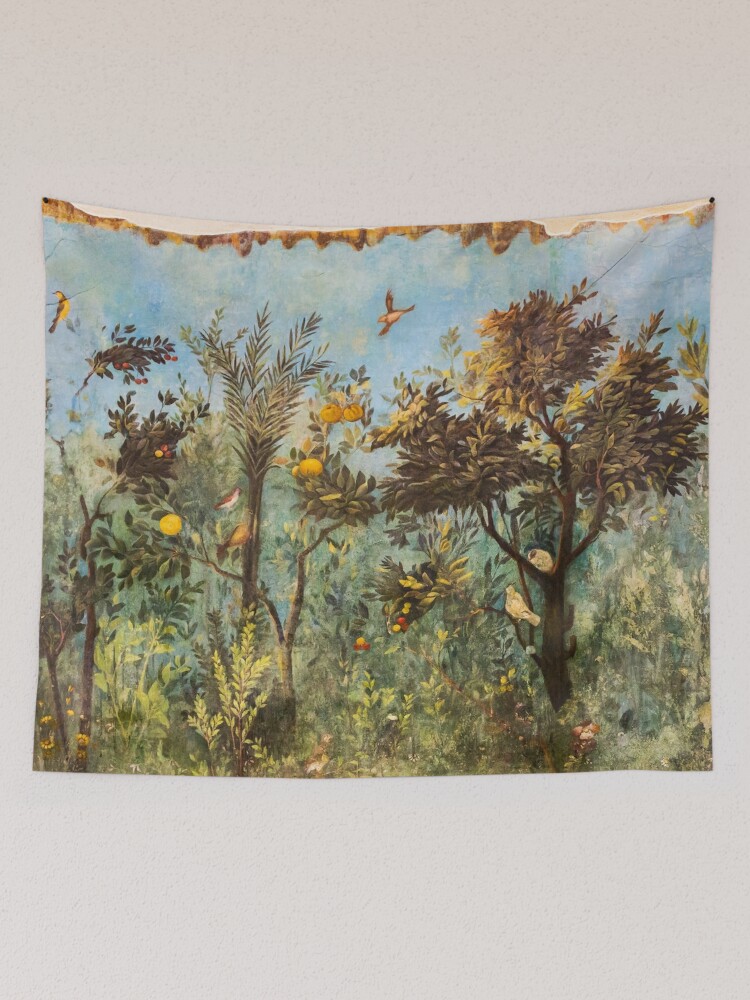This image displays a detailed nature scene painted on a fabric-like material, hung on a pale tan or grey wall. The fabric itself exhibits slight droops on either side, indicating its cloth-like texture. Dominating the scene is a vibrant blue sky, speckled with clouds and traversed by two birds—one with a yellow belly and possibly a woodpecker to the left. The landscape below is lush and varied: to the right stands a grand tree, home to a white bird perched on a branch and a possible bird's nest nestled in its crook. Adjacent, a smaller, thin tree with sprawling branches is dotted with what could be bird nests. To the left, another type of tree reaches upwards, decked with blooms and possibly oranges or yellow fruits akin to lemons. The scene's base is a verdant expanse of marshy foliage, taller weeds, and shrubbery, interspersed with light green plants and small clusters of orange and red berries. This rich tapestry of plant life and wildlife captures the essence of an untamed outdoor wilderness.